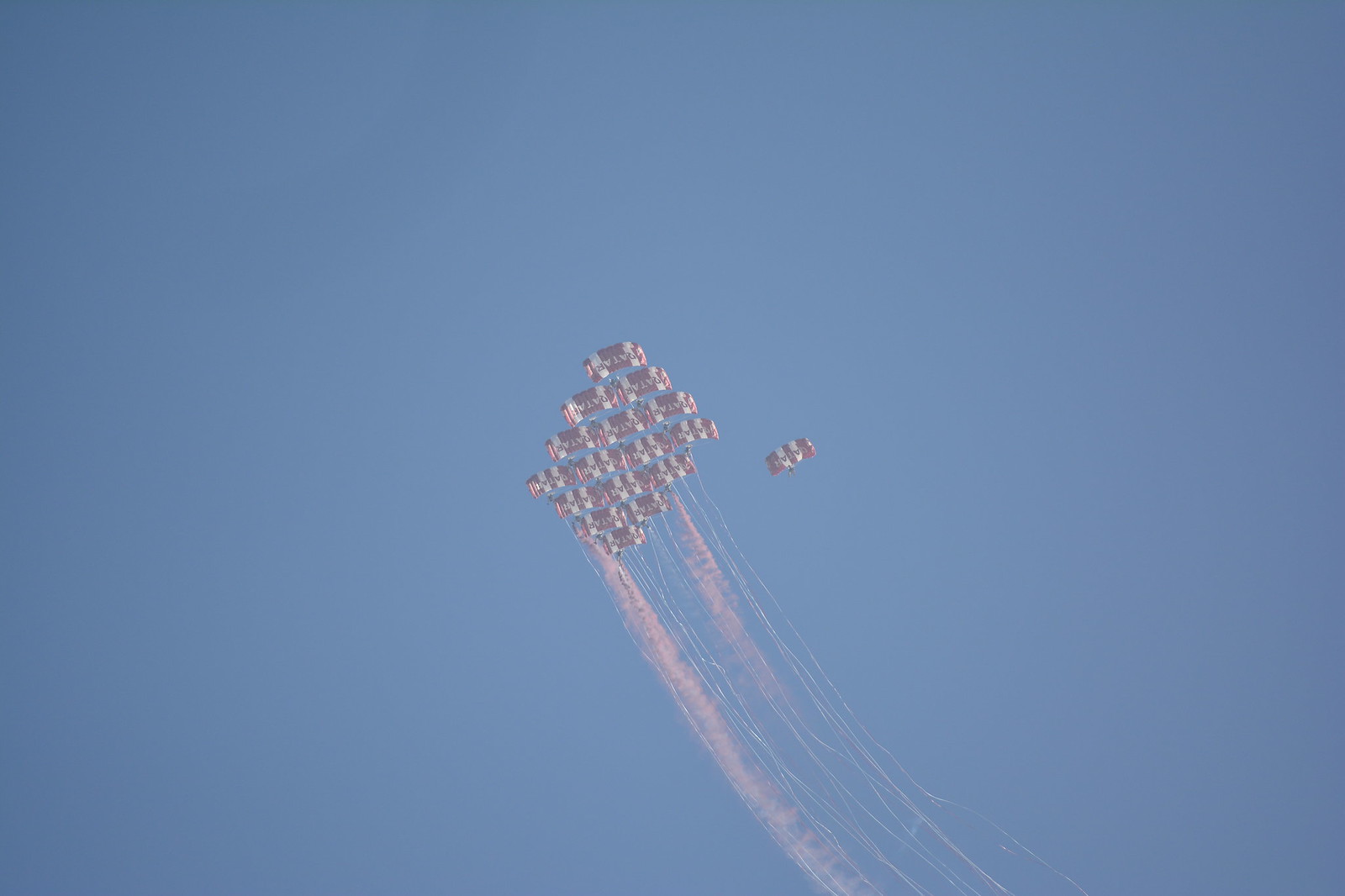The photograph showcases a vibrant, clear blue sky with a striking formation of 16 red-and-white striped rectangular parachutes at the center. These paratroopers are arranged in a diamond-like 4x4 grid formation. Thin white trails and a couple of thicker pinkish smoke trails extend from the cluster, emphasizing their dynamic descent. One additional parachute can be seen slightly to the right of this main formation. The perspective suggests the photographer is directly below, capturing the pristine blue sky and the dramatic display of colors and geometric precision.